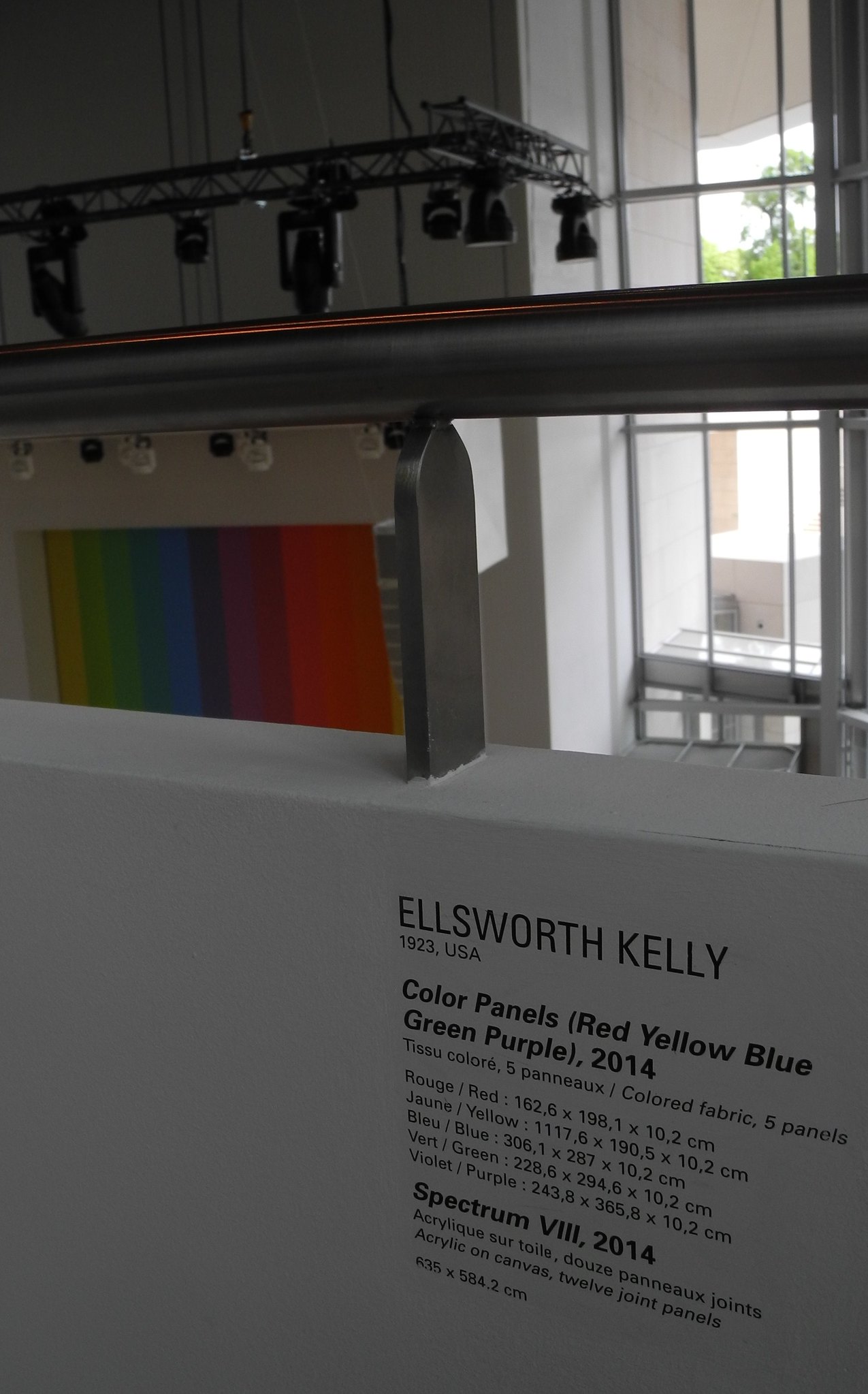This portrait-oriented color photograph captures an interior view of a museum, taken from a balcony overlooking a vibrant piece of artwork. The setting features a white boundary wall topped with a black metallic railing. Beyond the railing lies the rest of the museum, including various walls, windows, and a prominently displayed rainbow-colored poster. To the right on the white wall, black screen-printed text reads, "Ellsworth Kelly 1923 USA" followed by, "Color panels (red, yellow, blue, green, purple), 2014." Below is detailed technical information about the artwork, including dimensions and materials, with references to "spectrum VIII, 2014." The exhibit, spotlighted by overhead lighting on a metal framework, presents a partial view of multi-colored striped canvas panels mounted on the wall below, adding to the overall vibrant and artistic atmosphere.